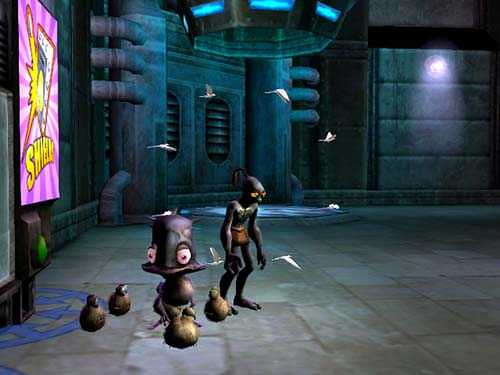This image appears to be a digitally rendered still from a video game, set inside a dimly lit, industrial interior. The environment features a dark gray tile floor and walls that are cluttered with pipes, vents, and conduits, creating a gritty, mechanical atmosphere. Toward the right of the scene, there's a billboard with a bright pink and purple background and yellow text, although the text remains partially obscured due to the angle. In the center of the image stand two distinct figures: one is a hunched, human-like creature with a bulbous head and large yellow eyes, wearing a dark, wetsuit-like outfit; the other figure resembles a non-human organism with a bell-shaped head, large eyes, and possibly four legs, also covered in a similar suit. Between them are four bird-like creatures with rounded bodies and heads, possibly robots given their simplistic, ball-like forms. The focal area is surrounded by a circle of white birds in mid-flight, enhancing the dynamic nature of the scene. To the side of the human-like figure, there appears to be a brown pack or accessory, while the non-human creature is accompanied by a robot that has big white eyes and a top hat-shaped body. The overall scene exudes a sense of otherworldliness and technological complexity, evocative of a richly detailed video game environment.